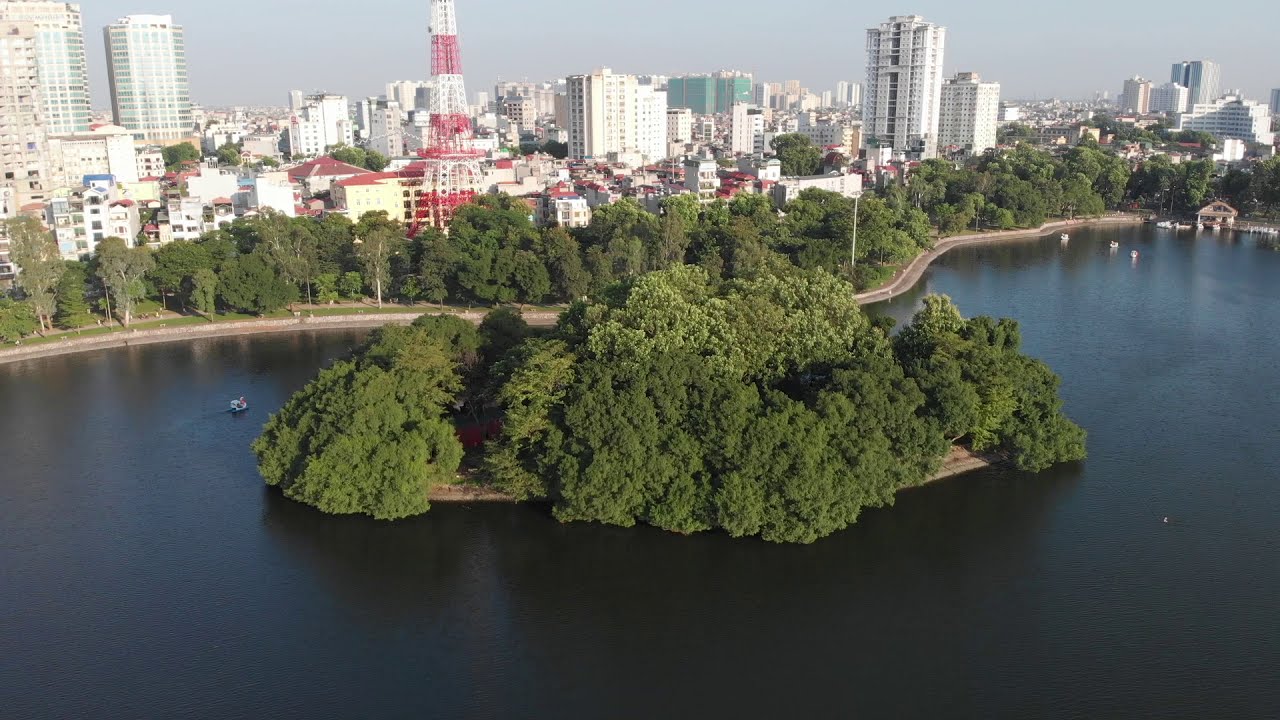An aerial daytime view reveals a serene bay with strikingly dark blue, almost black, still waters. Nestled within the bay is a small, lush island teeming with dense, bushy foliage, possibly hiding a shadowed red house. Along the upper half of the image, a walkway bordered by an abundance of green trees curves around the water’s edge. This scenic pathway leads to a bustling city backdrop, dominated by numerous white buildings, some rising as high as 30 stories. Among these structures stands a distinctive red and white striped metal tower, reminiscent of the Eiffel Tower, albeit shorter. The lake area is dotted with multiple paddle boats, adding a touch of activity to the tranquil setting. Overall, this vibrant image features a range of colors including greens, whites, reds, and the deep blues and blacks of the water, capturing a picturesque blend of natural and urban landscapes.